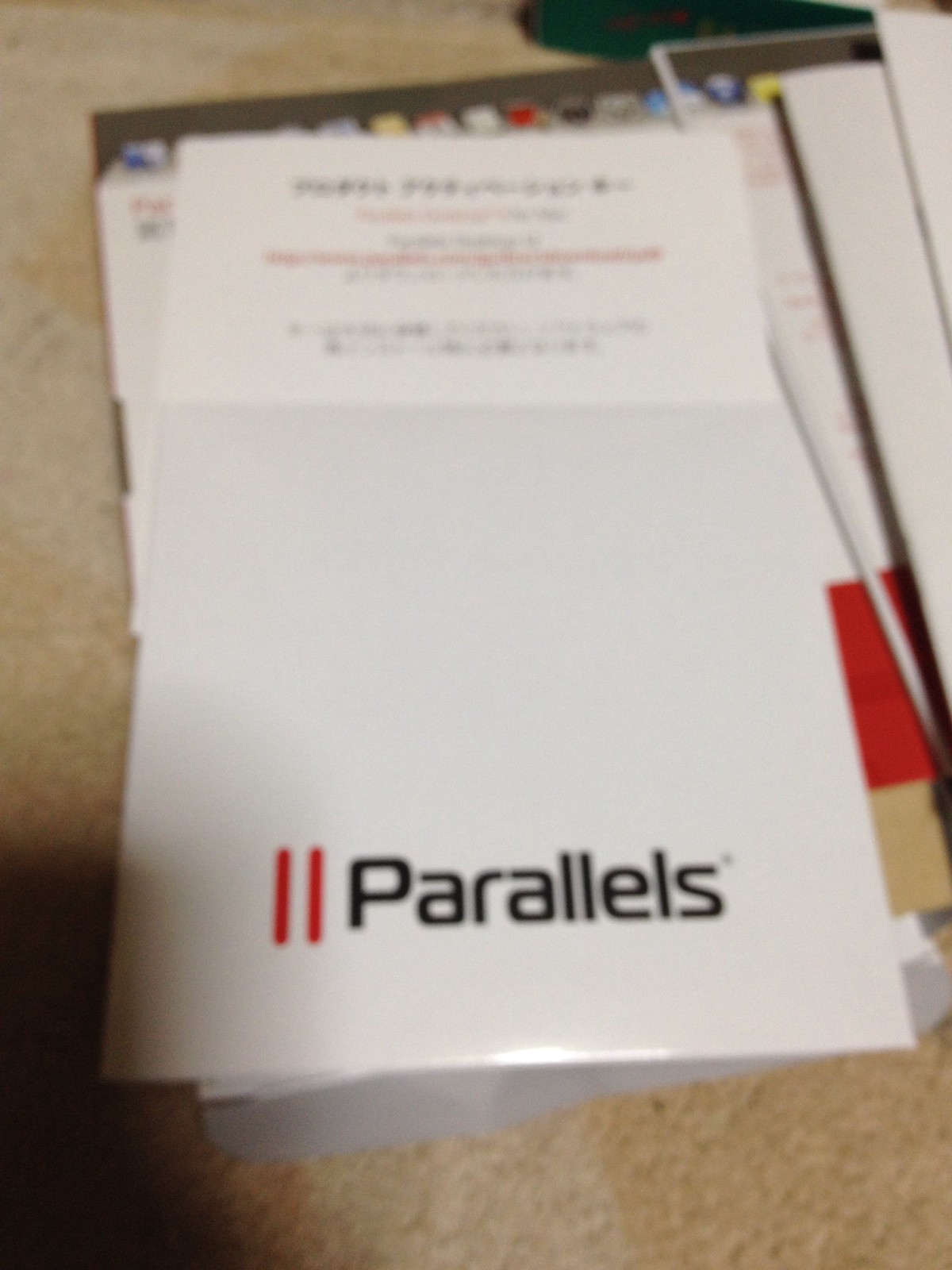The image showcases a slightly blurry scene dominated by a rectangular white piece of thick, laminated paper. Occupying the top third of this paper is a centered block of text with both black and red writing arranged in horizontal lines; however, the blur makes the text illegible. Extending to the bottom half of the image, two vertical red parallel lines are noticeable. To the right of these lines, the word "Parallels" is written in black with a capital 'P', and a faint symbol, possibly a trademark symbol, hovers above the 'S'. Beneath this primary paper, there appears to be an organizer, suggested by the visible edges of surrounding papers and hints of colored tabs at the top. The entire scene rests on a light brown or tan surface, with a noticeable dark area in the bottom left corner suggesting the shadow of the person who captured the image.